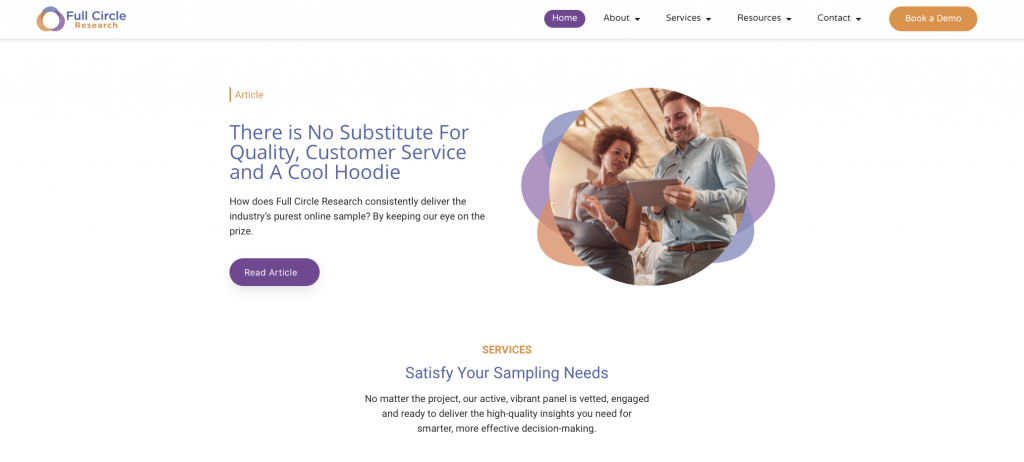The image is a detailed screenshot of the homepage of the "Full Circle Research" website. The background of the page, including the header, is white. On the left side of the header, the company's name, "Full Circle Research," is presented: "Full Circle" is in bold purple font, while "Research" appears in a smaller orange font beneath it. To the left of the company name is their logo, which resembles a three-petaled flower created with intertwining purple and orange circles.

In the center of the header’s menu, there is a purple rectangular button with rounded corners labeled “Home” in white text. The other menu items—"About," "Services," "Resources," and "Contact"—are written in gray with small inverted triangles next to each, indicating dropdown menus. On the far right of the header is an orange rectangular button with rounded corners, saying “Book a Demo” in white text.

Separating the header from the main content of the webpage is an extremely thin lavender-colored line. In the center of the page, there is an article title and descriptor. The word “Article” is written in small orange font, followed by the main title in purple, proclaiming, “There is no substitute for quality customer service and a cool hoodie.” Beneath this, a sentence in standard black font reads, “How does Full Circle Research consistently deliver the industry’s purest online sample? By keeping our eye on the prize.” Below this text is a purple rectangular button with rounded corners that says “Read Article” in white font.

To the right of this text block is a circular photograph featuring two individuals. On the left is a medium to light-skinned Black woman with short, reddish-brown natural hair. Next to her stands a taller white man, approximately in his 30s, with brown hair. He is wearing a blue shirt and holding a tablet, possibly an iPad, and they are both engaged, looking at the screen.